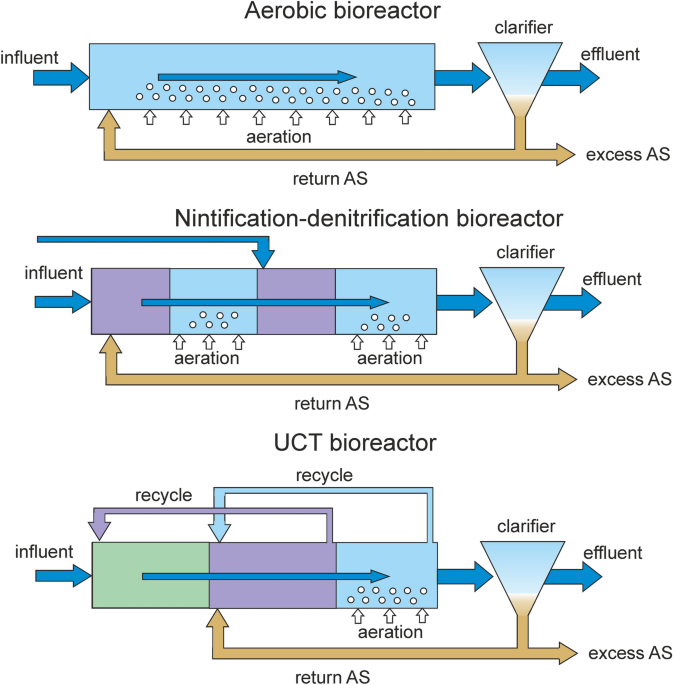The image is a composite diagram illustrating three different types of bioreactors, each processing influent and producing effluent and excess. The diagrams are stacked vertically with the influent shown on the left and the effluent and excess on the right. The top diagram, labeled "Aerobic Bioreactor," is primarily blue in color. The middle diagram, labeled "Nitrification-Denitrification Bioreactor," also showcases a similar color scheme with flow arrows indicating processing steps. The bottom diagram, labeled "UCT Bioreactor," features a unique green-colored box in addition to the blue design. All diagrams share common features, including arrows showing flow direction, aeration, return AS, and excess AS, which are marked with gold labels at the bottom. This comprehensive visual layout demonstrates the different steps involved in each bioreactor's treatment process.